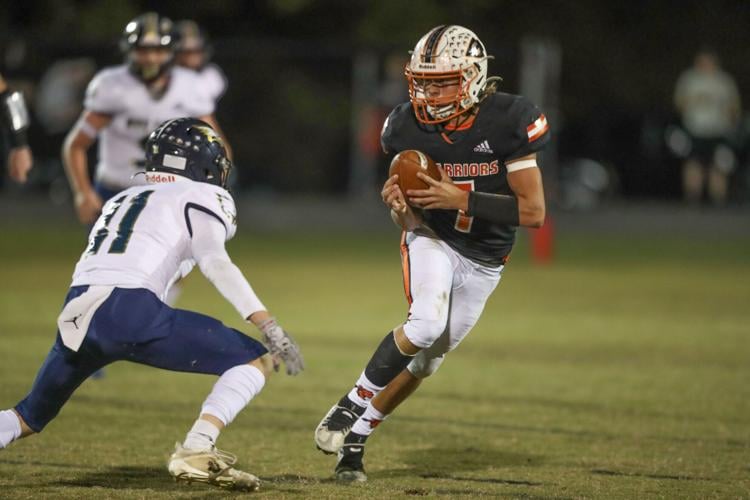The image captures a dynamic moment in a football game, likely at the minor league or high school level, featuring two central players. The focal player, donned in a black Adidas jersey with "Warriors" emblazoned on it and the number 7 in a reddish-orange hue, is holding the ball as he slants away from a defender. His attire includes white pants with a matching reddish-orange stripe, white cleats, white socks with a red emblem, a white armband around his bicep, and a black wristband. He sports a white helmet with a red face guard.

The opposing defender, captured with his back towards the camera, wears a white jersey that features an eagle logo, paired with purple pants. He is number 11, and the back of his helmet displays the name "Riddle." This player also has a blue helmet and white sneakers. The flat, green field further highlights the players, while background figures—other players and possibly coaches or spectators—blurred at the sidelines, actively watch the unfolding play.